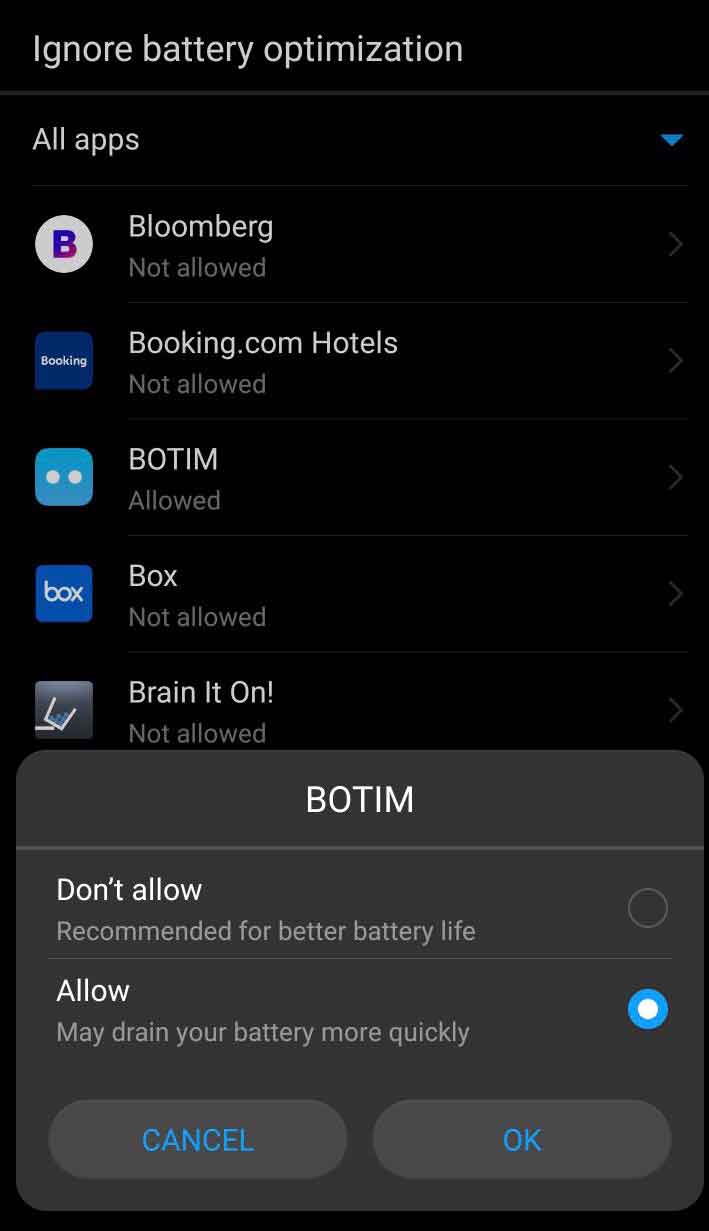The image showcases a smartphone screen displaying the settings section for app permissions and battery optimization. The background of the page is black, creating a stark contrast with the white text for improved readability. 

At the top of the screen, a header reads "Ignore battery optimization." Below this, the text "All Apps" indicates that the list pertains to the battery optimization settings for all installed applications. 

The following apps and their respective permissions are listed vertically:
- Bloomberg: Not Allowed
- Booking.com: Not Allowed
- Hotels: Not Allowed
- BOTIM: Allowed
- Box: Not Allowed
- Brain It On: Not Allowed

Further down, a pop-up appears in a square shape with rounded corners. The pop-up has a grayish background, and in the center, white text provides options for the BOTIM app. It reads, "BOTIM" followed by options "Don't Allow" and "Allow." The "Allow" option is selected on the right side, with a note indicating, "May drain your battery more quickly." Additionally, there are "Cancel" and "OK" buttons at the bottom of the pop-up.